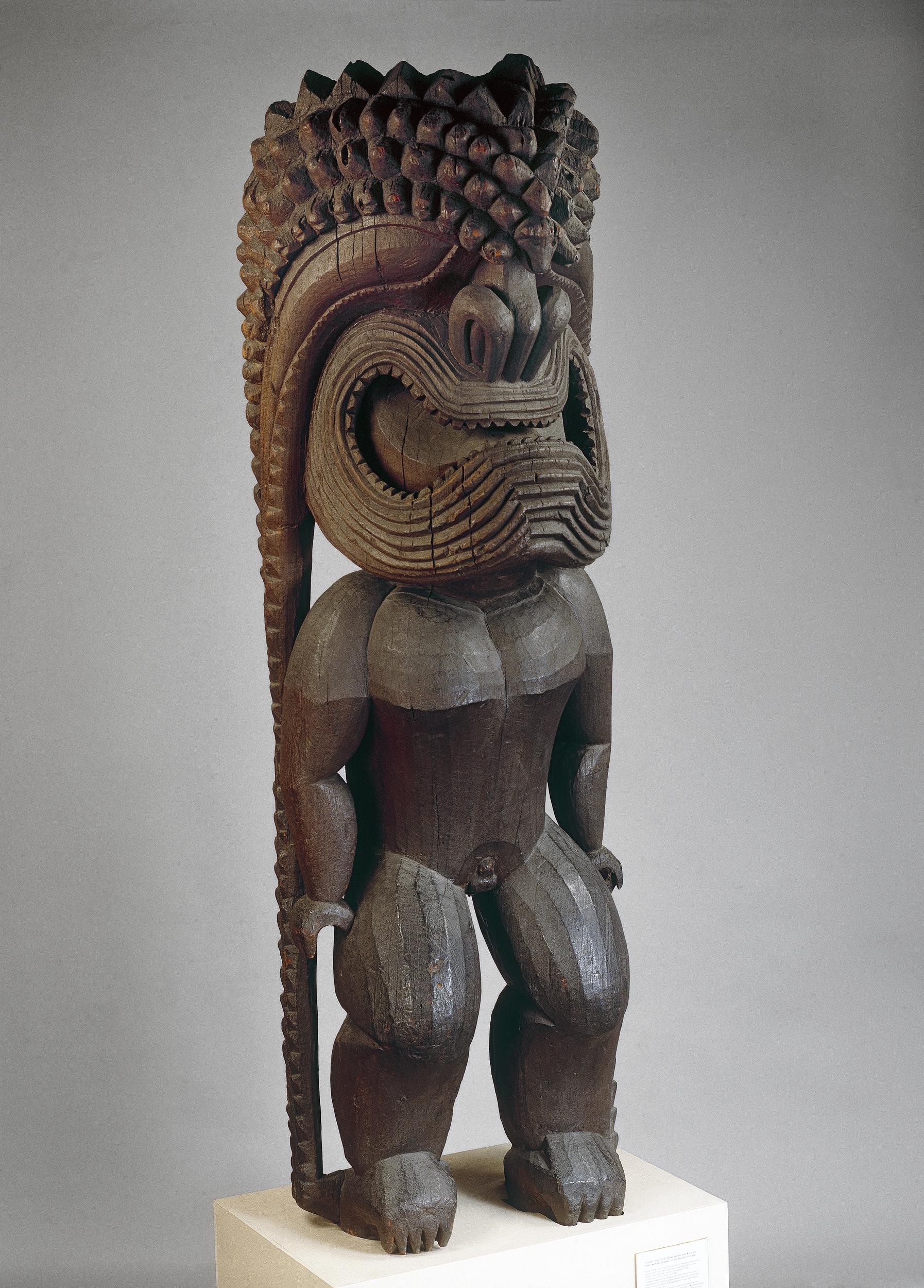This is a detailed photograph of a traditional, dark wooden statue displayed in a museum setting against a plain gray wall. The statue stands on a white or off-white square cuboid display stand. The figure is unclothed, revealing exposed genitalia, and features a muscular chest with thick legs, though its fingers and toes are minimally detailed and pressed in.

The statue's head is notably large compared to its body, almost as tall but slightly shorter, and adorned with long, ridge-like hair that extends from the head down to the feet, resembling a dragon’s tail. The head itself resembles a tribal mask, with large eyes, a prominent nose, and a grimacing mouth that is open wide, almost as if placed where human eyes would be. This headpiece lends the figure an almost mask-like appearance, which some believe to be reminiscent of South American tribal masks, though its exact cultural style is uncertain.

Though the statue's body is a dark brown wood and lacks any accent colors or paint, different sections exhibit slight variations in hue, possibly indicating the original artist’s intention to show clothing or adornments. The stance of the figure is upright and passive, simply standing still, as if silently observing its surroundings.